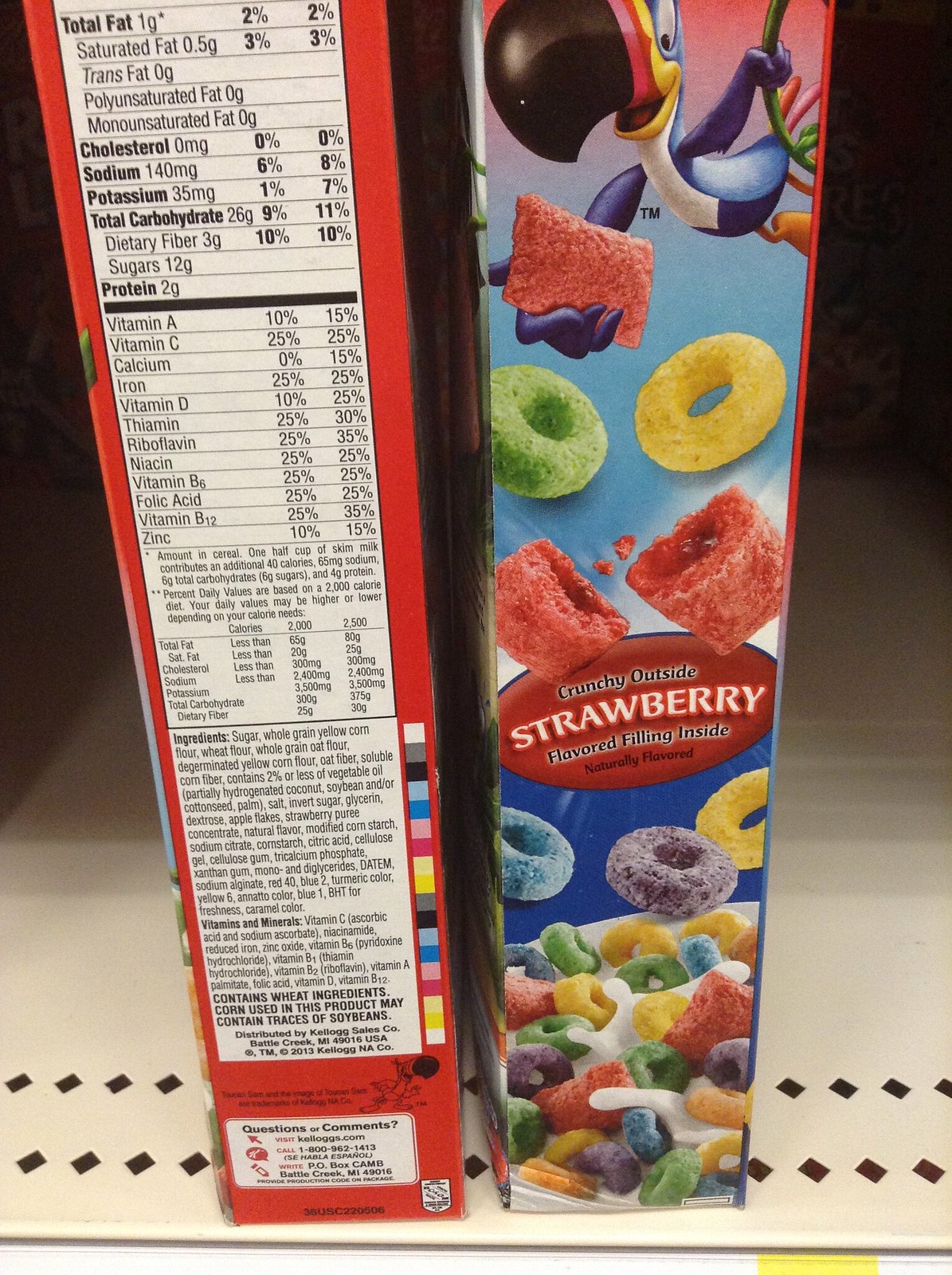On a shelf, there are two boxes of Froot Loops cereal. The box on the right prominently features Toucan Sam at the top. Toucan Sam has a large black beak and a colorful face with shades of pink, red, and yellow, while his body is blue with multicolored tail feathers. One of his feet is orange, and his right hand is holding a pink square object. Below this, there is a depiction of a red object, which appears to be cracked in the middle, along with the text stating "Crunchy outside, strawberry-flavored filling inside." Surrounding Toucan Sam are colorful loops in various shades: yellow on the right, green on the left, and a blue, purple, and yellow loops at the bottom.

There is also an image of a bowl of cereal filled with white milk and numerous colorful loops. To the left of the artwork is the nutrition facts panel, which lists total fat, cholesterol, sodium, potassium, vitamins (A, C, D, thiamin, riboflavin, niacin, B6, B12, folic acid), calcium, iron, and zinc. At the bottom of the panel, the ingredients are listed, which include sugar (noted as the most prominent ingredient), whole grain, yellow corn flour, wheat flour, and brown flour. The box's primary colors are white, gray, black, light blue, blue, pink, red, yellow, and dark red.